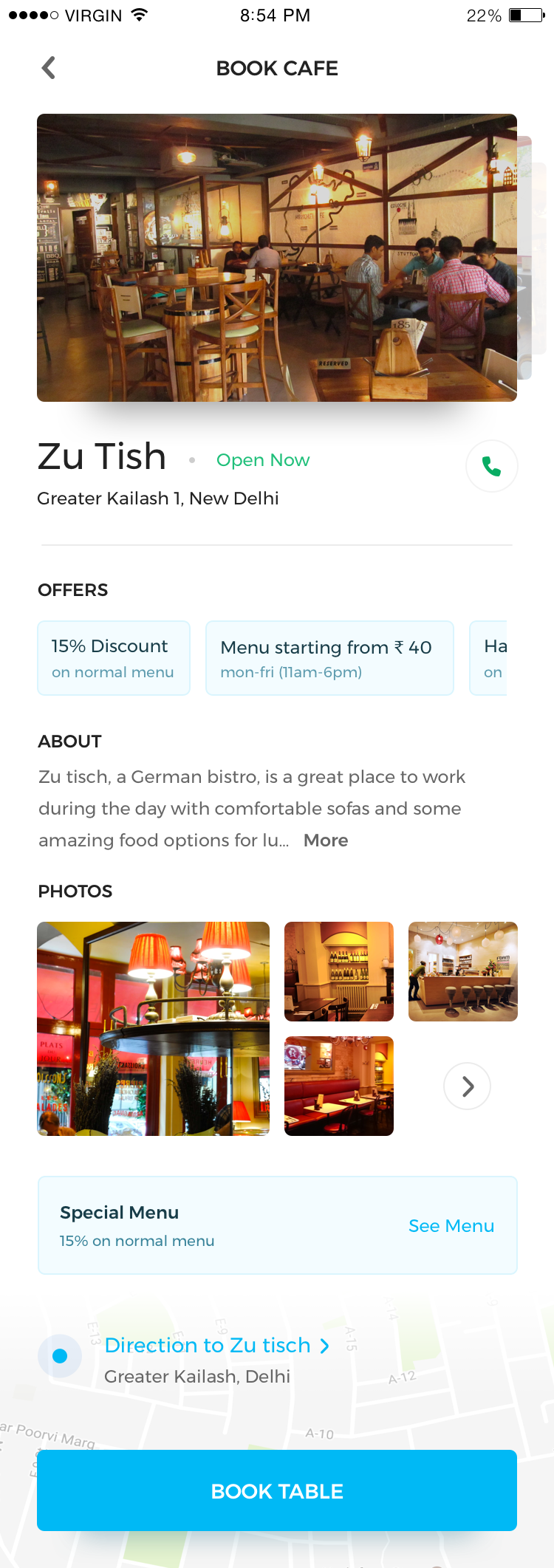**Caption for the Image:**

The image showcases a smartphone interface, reflecting various details about a cafe named Zoo Tishik in Greater Kailash 1, New Delhi. The top-left corner displays four black dots and a clear white dot, along with a 'Virgin' signal indicator and a Wi-Fi logo. The time reads 8:54 PM with a 22% battery life shown on the right.

Below, there's a navigation arrow pointing left, followed by the text 'book cafe' in the middle. The background is a warm brown-orange with yellow lights adorning the top, capturing the cozy ambiance of the cafe where people are seated and enjoying their time.

In black text, it says "Zoo Tish," followed by "Open Now" in green font, and an icon of a green phone in a grey circle. The address "Greater Kailash 1, New Delhi" appears beneath it. A grey line precedes the section on offers, listing a "15% discount on Normal Menu" available from Monday to Friday, 11 AM to 6 PM, against a light blue background.

An 'About' section describes Zoo Tishik as a German bistro ideal for working during the day with comfortable sofas and diverse lunch options. This is followed by a 'Photos' section showing four images, the first depicting orange lamps, enhancing the cafe's aesthetic.

A grey circle with an arrow inside appears below the fourth photo. The 'Special Menu' section stands out with a blue background, offering a 15% discount on the Normal Menu, and a 'See Menu' option to the right. Lastly, a map shows the cafe’s location, with a grey base, green patches (indicating parks or similar areas), and white lines (representing streets). Directions to 'Zoo Tish' are highlighted, accompanied by a 'Book Table' button in a blue box with white lettering.

Overall, the snapshot provides comprehensive information about the cafe, including its menu, ambiance, and location, aimed at enticing potential visitors.